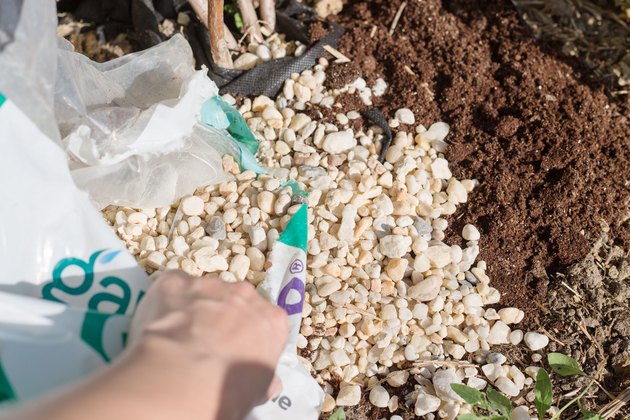A close-up image shows the back of a white Caucasian person's hand as they rip open a white plastic bag adorned with green lettering. Scattered around the freshly torn bag are jagged shards of white plastic. The contents, resembling small white rocks or pebbles, have spilled onto the soil below. The soil in the foreground is light and fluffy with a brown hue, transitioning to a greenish-gray patch towards the right side of the image. In the bottom right corner, a touch of greenery can be seen, possibly leaves or weeds. It appears the person is spreading these white pebbles over the soil, possibly for use as ground cover in a garden or similar outdoor project.